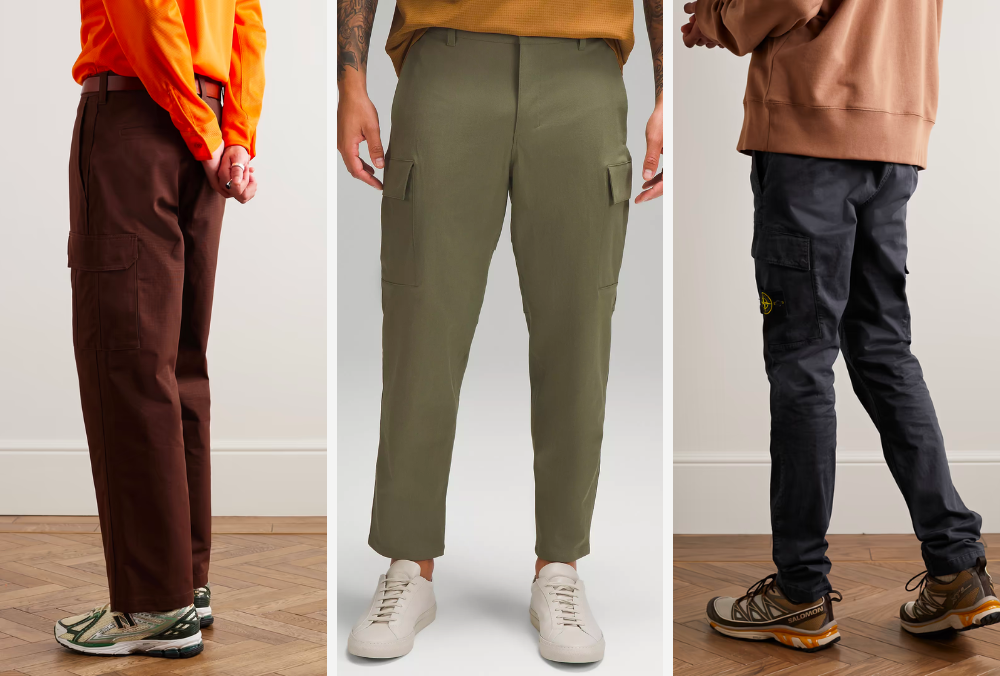The image presents three juxtaposed photos, each showcasing a male model wearing different pairs of pants. The leftmost photo displays a model in brown cargo pants with prominent side pockets, paired with an orange long-sleeved shirt and a brown belt. He stands against a white-walled background on a white wooden floor, sporting New Balance tennis shoes in forest green, lighter green, and tan. Notably, his hands are clasped behind his back, adorned with rings on his thumb and pointer finger.

The center photo features a close-up shot from the waist down of a model donning green cargo pants with large pockets on both thighs. He wears white shoes and a mustard-colored short-sleeved t-shirt. His forearms, which hang naturally at his sides, are tattooed. The background is consistent with the previous photo.

In the rightmost photo, the model is depicted wearing black or navy blue cargo pants with side pockets, accompanied by an orangish-peach long-sleeved sweatshirt, which might be a hooded sweater. His slightly lifted right foot suggests a dynamic pose, facing away from the camera. His shoes are multi-colored—yellow, white, gray, and tan—resembling trail running or hiking shoes. Again, the background matches the clean, minimalist setting of the first two images.